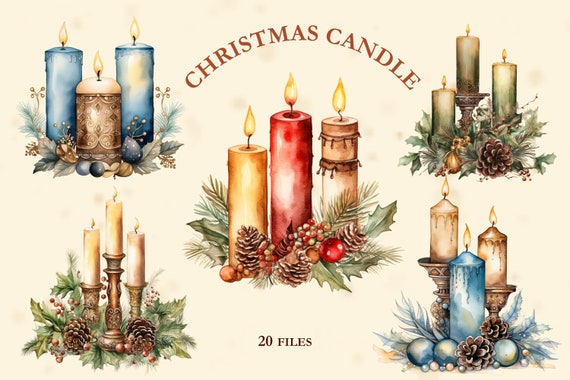This digital poster styled like a postcard features five different sets of Christmas candle displays. The central design showcases three lit candles—red, yellow, and tan—ascending in height and surrounded by a wreath of pine cones, acorns, and red holly berries. The title "Christmas Candles" appears prominently in dark red or brown print over a tan backdrop. To the upper left, there are blue candles, one held in an iron candle holder, accompanied by an arrangement of twigs, leaves, and berries. Similar groupings of trios of candles in gold and other festive colors appear at the upper right and lower right, each adorned with Christmas decorations such as pine cones and holly. The text "20 files" in black lettering is included in the middle, suggesting a collection of 20 different designs or arrangements.